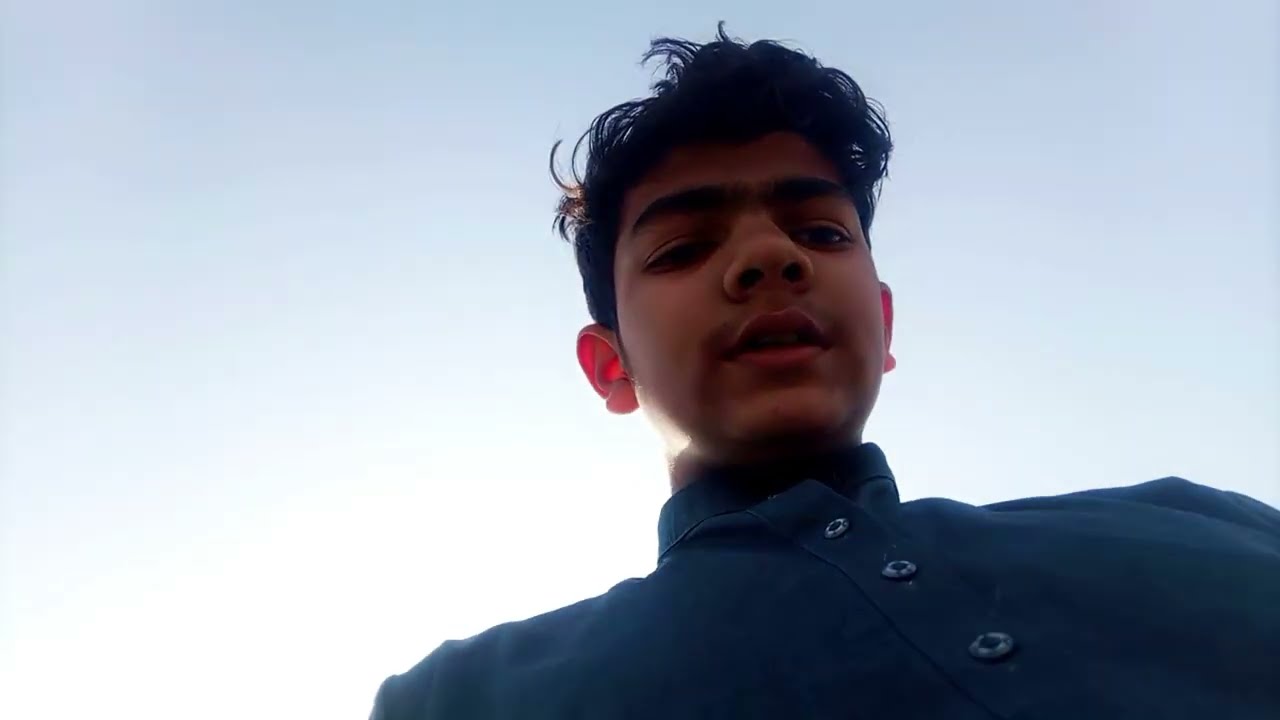This photo-realistic image captures a selfie of a young man, possibly in his late teens, with brown skin and dark, curly hair. He has striking dark eyebrows and brown eyes. He is adorned in a blue button-up, collared shirt, distinguishable by three buttons at the center. The image is taken from a low-angle perspective, providing a view from below him, slightly off-centered to the right. The young man's expression is neutral, and although he seems to be talking, his exact emotions are indistinguishable.

The background is predominantly a clear sky, transitioning from a light blue at the top to bright white at the bottom left corner. The selfie is backlit by the sun, casting the young man in shadow and giving a clear, outdoor daylight setting without any text or additional objects in the view, reflecting a typical scene you might encounter on social media.